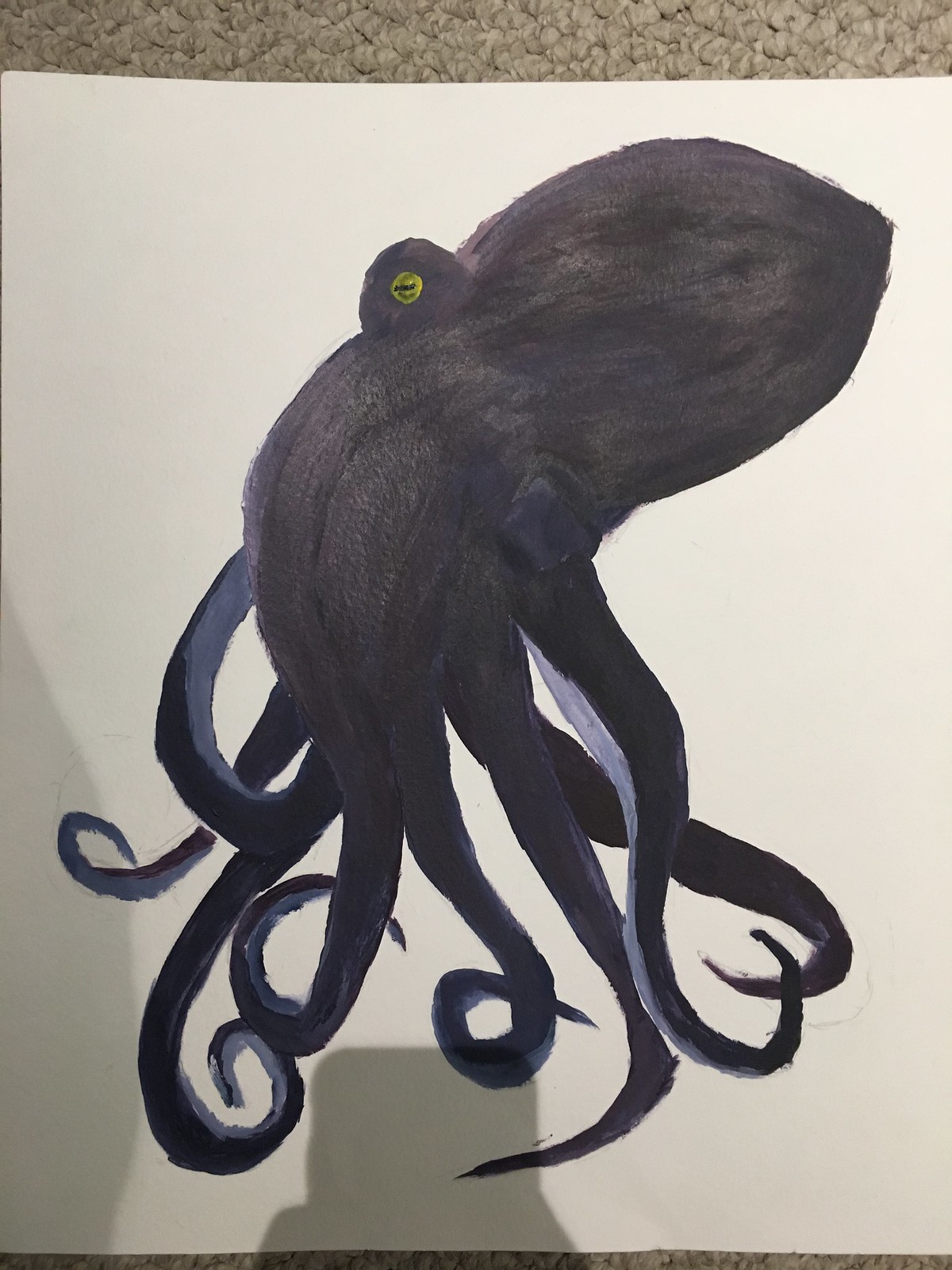The image showcases a meticulously painted marine creature, possibly an octopus or a squid, against a white sheet of paper placed on a tan carpet. The creature's body and tentacles are rendered in rich black hues, with the inner surfaces of the tentacles delicately shaded in light gray. Its head, an oval shape, tilts slightly to the right and culminates in a subtle rounded point. Prominently, a round eye protrudes from the side of its head, featuring a striking yellow iris bisected by a black stripe. The front of the marine creature displays four tentacles extending downward, with their tips elegantly curling back upwards. The back side reveals an additional three to four tentacles, completing the dynamic and intricate depiction of the creature.